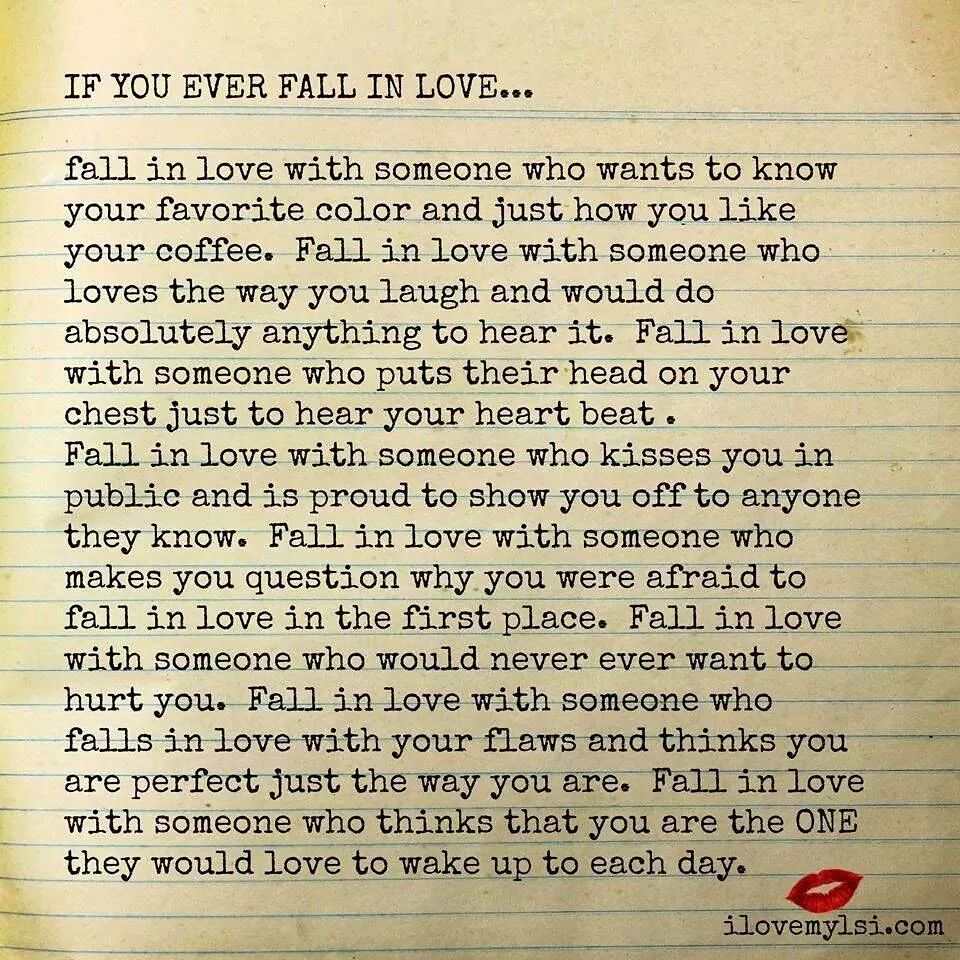The digitally created image features a poem set against a background resembling lined notebook paper, giving it a handwritten feel. The poem is in black text and appears to be computer-generated rather than actually printed on the paper. The text reads: "If you ever fall in love, fall in love with someone who wants to know your favorite color and just how you like your coffee. Fall in love with someone who loves the way you laugh and would do absolutely anything to hear it. Fall in love with someone who puts their head on your chest just to hear your heartbeat. Fall in love with someone who kisses you in public and is proud to show you off to anyone they know. Fall in love with someone who makes you question why you were afraid to fall in love in the first place. Fall in love with someone who would never ever want to hurt you. Fall in love with someone who falls in love with your flaws and thinks you are perfect just the way you are. Fall in love with someone who thinks that you are the ONE they would love to wake up to each day," with "ONE" emphasized in all caps. In the bottom right corner of the image, there is a URL that reads "IlovemyLSI.com" accompanied by an image of a red lipstick kiss, giving the image a touch of personality and intimacy. The text does not follow the lines perfectly, adding to the charm and casual feel of the poem.